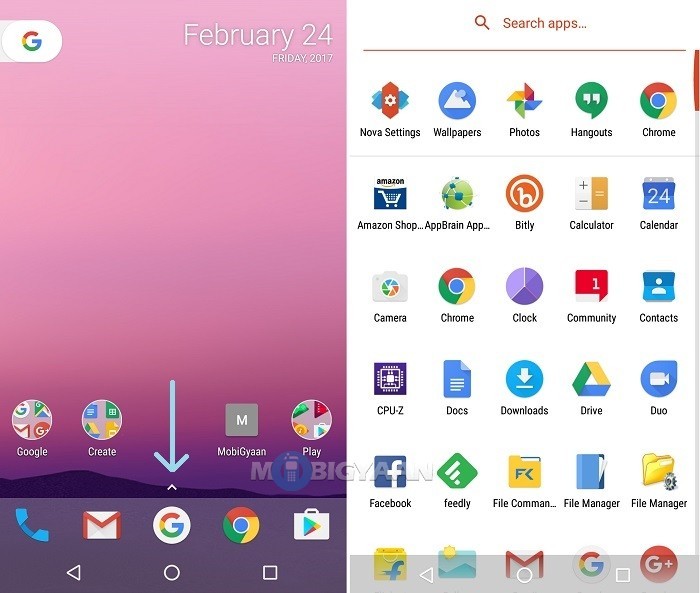A smartphone screenshot with a pink background prominently displays the date "February 24th, Friday, 2017" alongside a "G" for Google, indicating the use of Google services. The title "Google Create" is visible at the top, highlighting the image's association with Google functionalities. The app "MobiGyan" is mentioned, with "M" and "G" capitalized and presented as one word. The screen shows several core apps in a grid format, including icons for Search Apps, Nova Settings, Wallpapers, Photos, Hangouts, Chrome, Amazon Shop, App Brain, Bitly, Calculator, Calendar, Camera, Clock, Community, Contacts, CPU-Z (shown in all capital letters), Docs, Downloads, Drive, Duo, Facebook, Feedly, and what appears to be "File Command" partially displayed as "C-O-M-M-A-N dot, dot, dot," followed by File Manager shown twice. At the bottom of the screen, navigation icons are displayed: a left-pointing arrow, a circle, and a square, which are common Android device controls. The setup is organized into two screenshots side by side, both capturing an identical array of icons and navigation buttons, framed in a cohesive, clean layout typical of a personalized Android home screen.